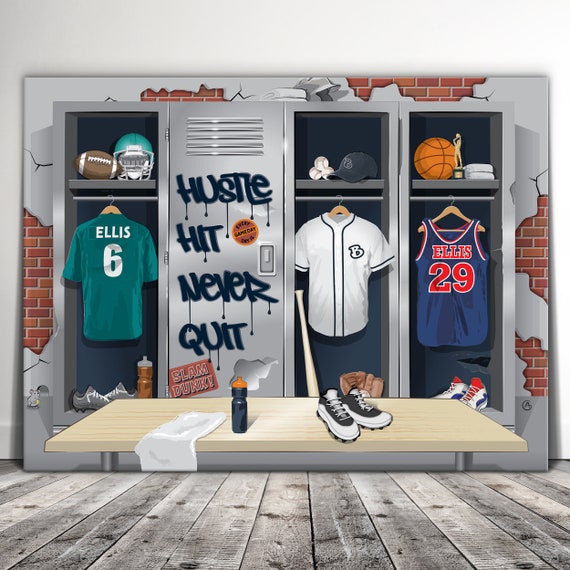This detailed graphic illustration of a locker room showcases a vividly designed environment. The backdrop features a distressed and broken cemented wall, revealing underlying brown brick patterns and giving the impression of an aged, gritty space. Centered against this rugged background are four steel gray lockers. The first locker on the left belongs to Alice, number 6, from the football team, containing a helmet, a football, a football jersey, cleats, and a water bottle on the top shelf. The second locker is closed and features graffiti reading "Hustle, Hit, Never Quit." The third locker, an open baseball locker, holds baseballs, a baseball cap on the top shelf, and a baseball jersey hanging inside. The fourth locker belongs to Alice, number 29, from the basketball team, with a basketball, an award trophy, towels, a blue and red basketball jersey, and shoes. In front of this line of lockers is a wooden bench placed on a flooring of gray wooden planks, displaying a sports shoe, a water bottle, and a white towel. The entire scene is encapsulated in a digital art style, blending the realism of sports gear with the gritty atmosphere of an old locker room.